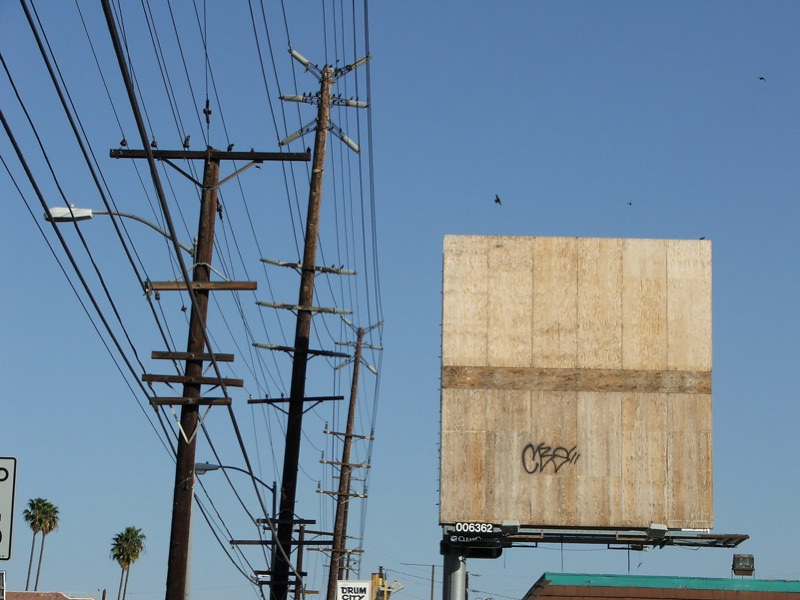In this rectangular photograph, taken from a low viewpoint looking up a street, the right side of the image features a large, double-tall wooden billboard devoid of any advertisements. The billboard is segmented into three colors: light tan on the top, dark brown in the center, and lighter brown on the bottom. It is covered in graffiti and has "CBDE" spray-painted in black on its surface. At the base of the billboard, the number 006362 is clearly visible. Adjacent to the billboard, a building with green trim can be faintly seen at the bottom of the image. 

Moving to the left side of the photograph, numerous telephone poles stand side by side, strung with a complex web of power and communication lines that stretch from the top left to the center of the picture. Below the tangle of wires, the bottom left corner reveals multiple palm trees situated in the distance, along with the edge of a black and white street sign. The background sky is a vivid blue, completely free of clouds, creating a striking contrast against the urban elements.